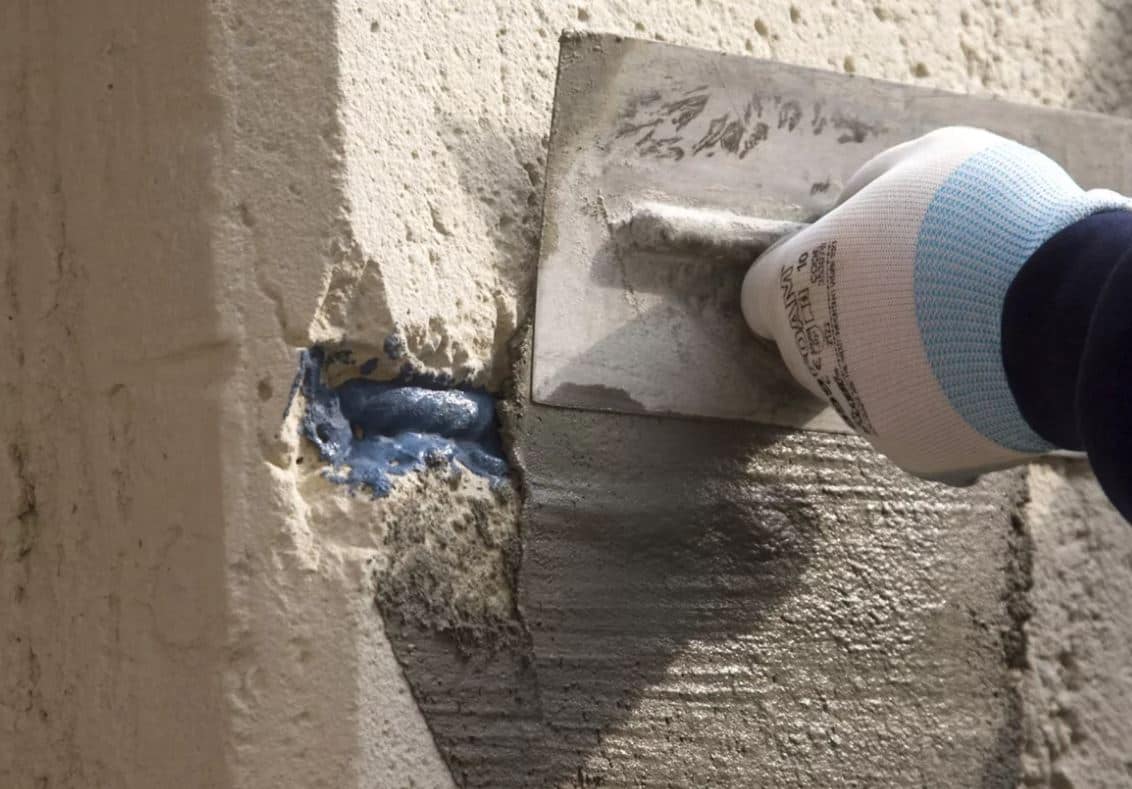The image captures a partially visible, tan-colored stone wall, imbued with historical texture and character. Embedded within this wall is a distinct piece of blue-painted metal, providing a vivid contrast against the earthy stone backdrop. A person’s left hand, adorned in a white glove with a light blue cuff, comes into focus as it grasps a metallic handle extending from the embedded metal piece. The glove, marked with indiscernible alphanumeric text, hints at either a function or identification. The metal handle, rectangular in shape and partially extending out of the frame, appears solidly attached to the wall’s upper right section. The overall composition leaves the viewer pondering the action being undertaken by the gloved hand, as the surrounding stone wall stretches towards the left and bottom edges of the image, emphasizing the scene's depth and intrigue.